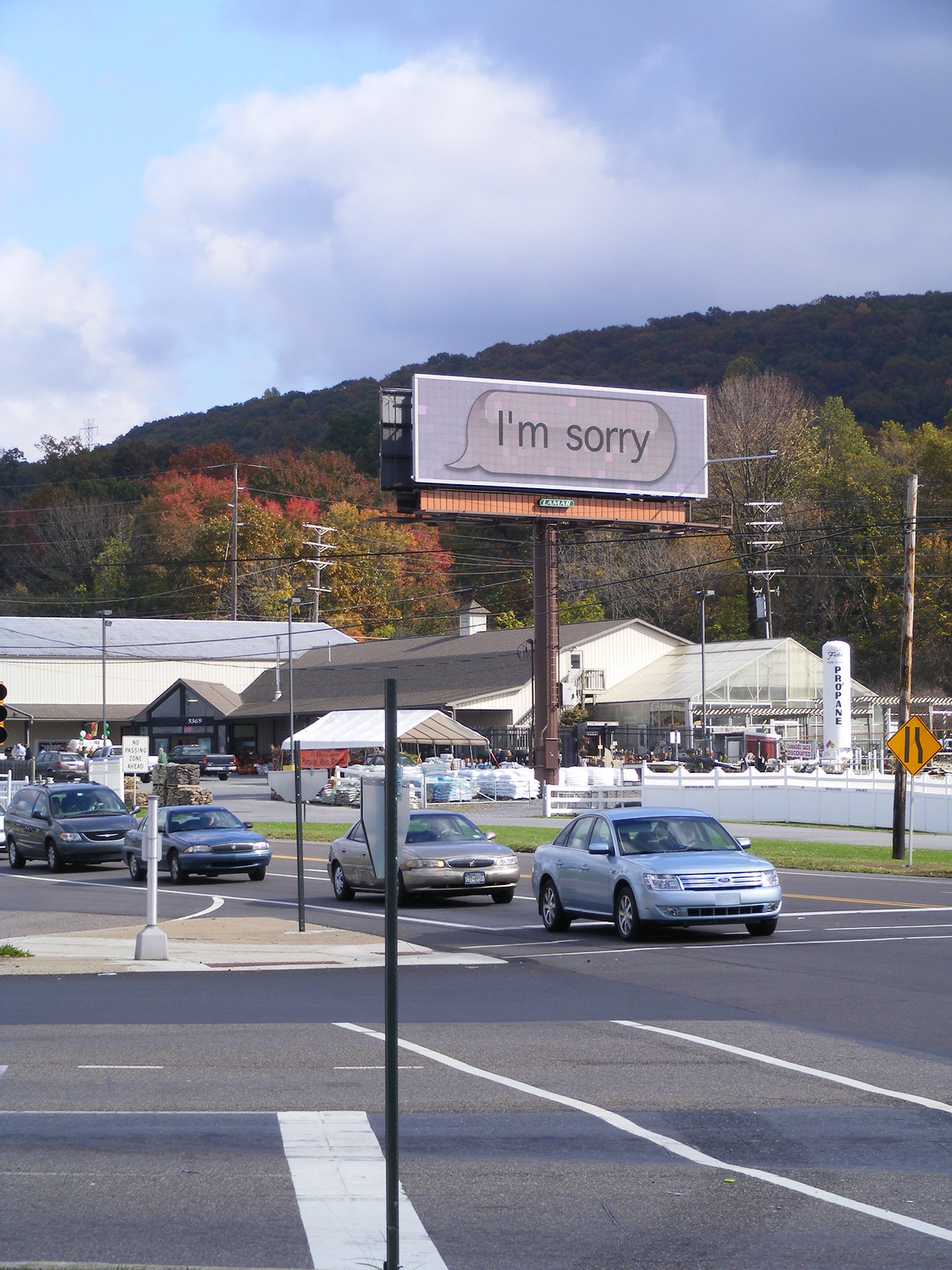This outdoor scene captures a bustling intersection in a quaint town, framed by a striking backdrop of mountains and trees adorned in vibrant autumn colors. In the background, a plaza houses several stores, including a prominent large building. Adjacent to the plaza, a small tent displays items for sale, suggesting a local market scene. The sky is a beautiful, expansive blue, dotted with fluffy white clouds. Four cars are lined up on the opposite side of the street, waiting to cross. A whimsical billboard with a comic-style word bubble reads, "I'm sorry," though it amusingly lacks a speaker. Telephone poles with crisscrossing wires add to the elements of small-town charm and connectivity.